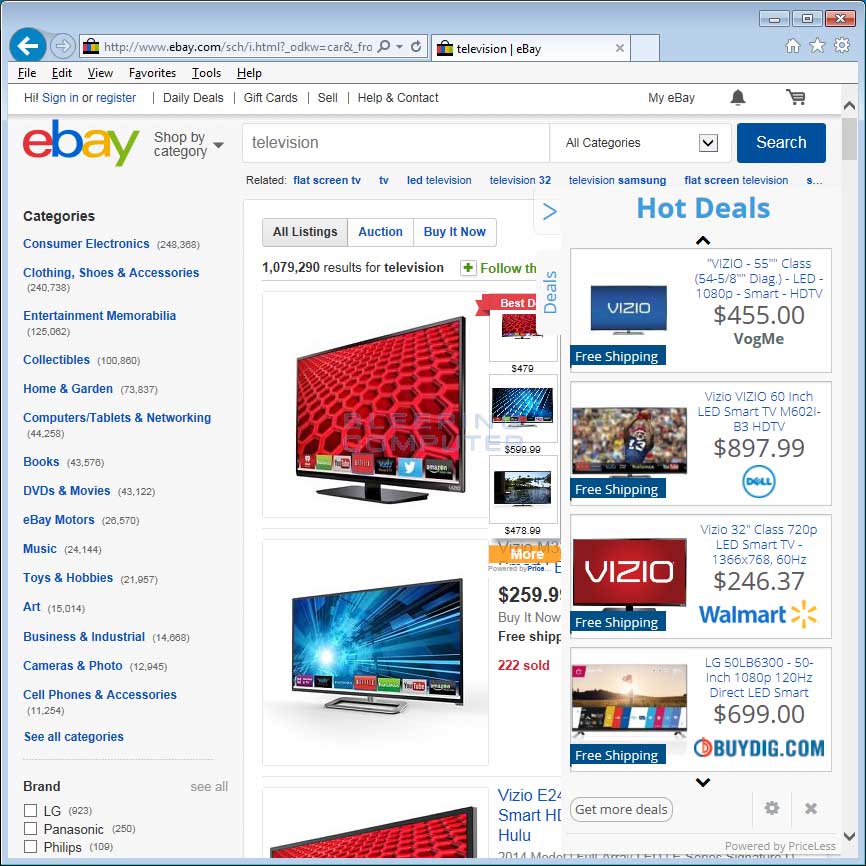The image depicts a web page from eBay, specifically featuring a selection of televisions. The browser tab prominently displays the word "televisions," indicating the user is browsing within this category. At the top of the page, there's an "X" button to close the website. Below the navigation bar, the eBay interface allows users to shop by category, with options clearly listed.

On the left side of the screen, a vertical sidebar presents various sub-categories related to televisions, each accompanied by the number of listings available. This filtering system enables users to sort through the products based on their preferences.

The main section on the right showcases a range of television sets, each item displayed with a thumbnail image and price. Particularly highlighted are "Hot Deals," offering discounted prices on selected TV models. This promotional section positions the latest offers prominently, enticing users to explore and potentially make a purchase.